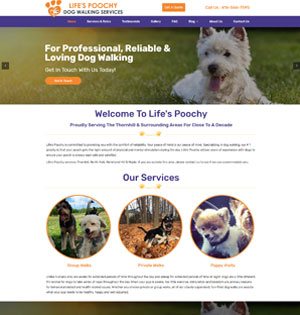This image is from the website "Life's Poochy Dog Walking Services," where "Poochy" is spelled P-O-O-C-H-Y. The website features a user-friendly layout with several drop-down menus; the first menu is highlighted in orange, while the subsequent seven are in white. Prominently placed at the top is an orange rectangle labeled "Get a Quote."

The image showcases a fluffy white Schnauzer-type dog lying contentedly on a lush, grassy yard, with its pink tongue playfully sticking out. Overlaying the grass is a caption in white text that reads, "For professional, reliable, and loving dog walking." Beneath this caption, there are additional words that are somewhat difficult to discern. 

Midway down the page, there is an orange button likely labeled "Start Now" or "Get a Quote." Continuing down to the middle section of the image, the text "Welcome to Life's Poochy" stands out. Below this greeting, more detailed information about the services is provided.

At the bottom of the image, under the "Our Services" section, three pictures of dogs highlight the various dog walking services offered by Life's Poochy.